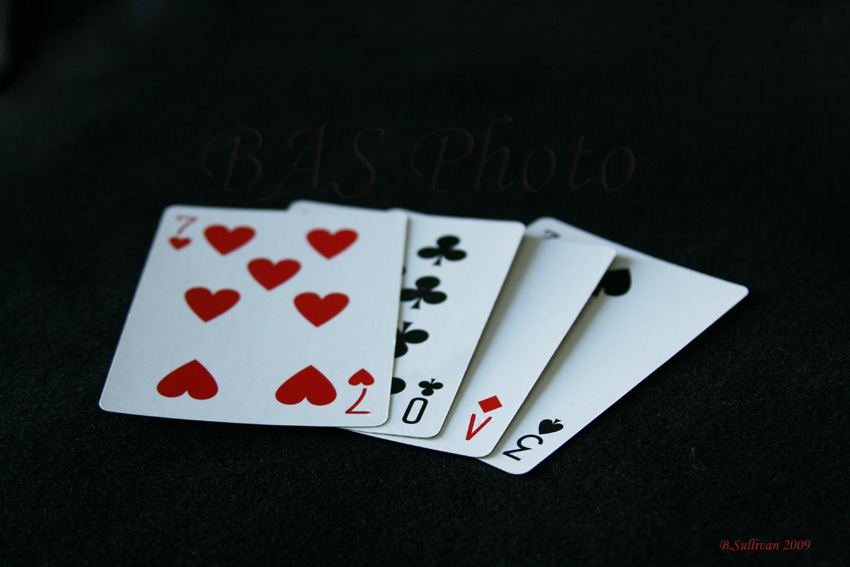In the image, four playing cards are arranged face-up against a solid black background. From left to right, the cards are a standard Seven of Hearts, a custom-designed Zero of Clubs, a custom V of Diamonds, and a standard Three of Clubs. In the bottom right corner of the background, there is a signature that reads "B. Sullivan, 2009." The custom cards add an intriguing touch to the otherwise conventional collection, standing out with their unique and non-traditional designs.